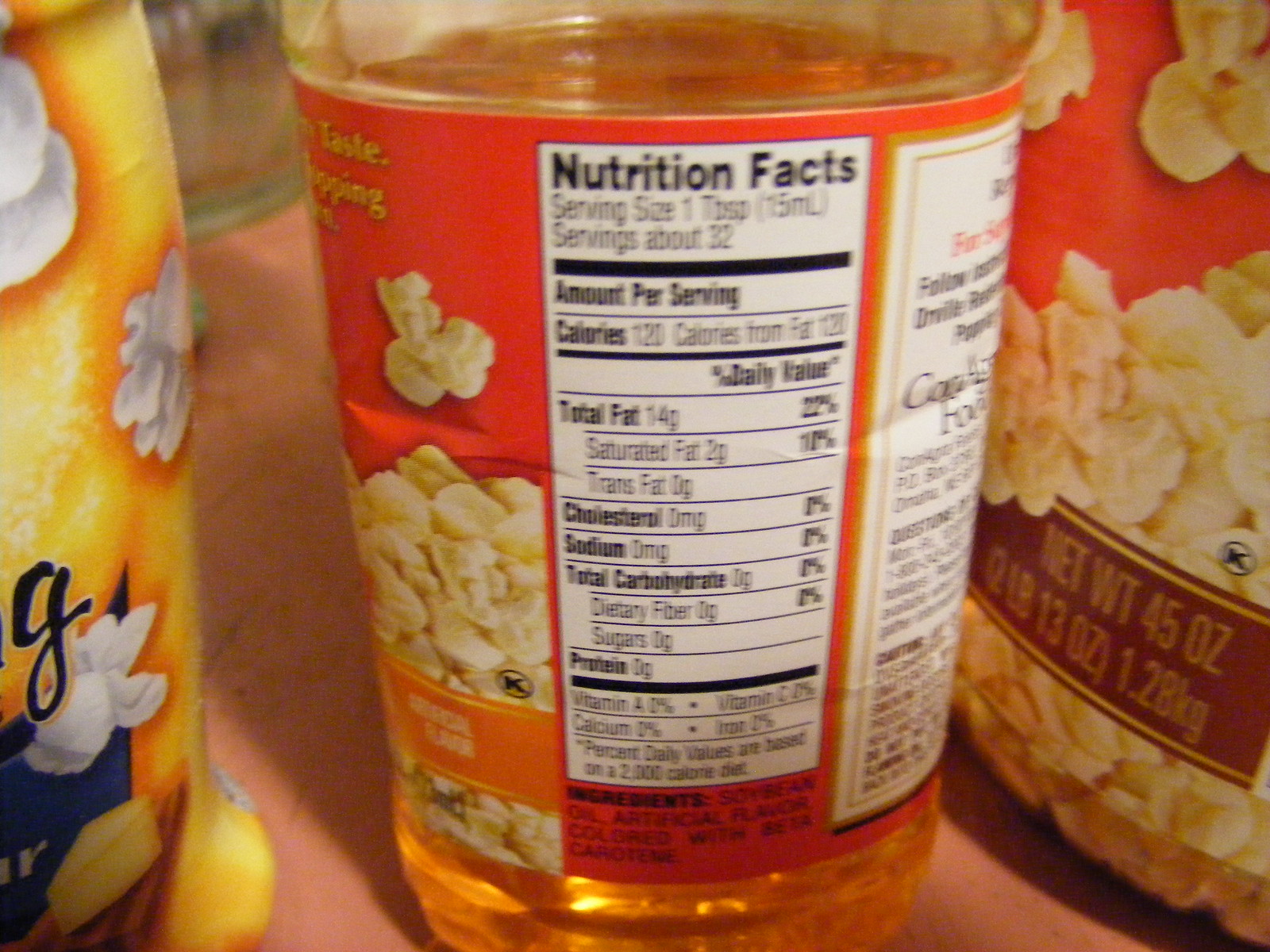The image is a close-up photograph showcasing several products on a light red or pink tabletop. Dominating the center is a transparent plastic bottle with an orange label, containing an orange liquid likely meant for drizzling on popcorn. The bottle's label prominently features nutrition facts, detailing a serving size of one tablespoon, 32 servings per bottle, 120 calories per serving—of which all calories come from fat. The total fat content is 14 grams, with 2 grams of saturated fat, zero trans fats, zero milligrams of cholesterol, and zero grams of total carbohydrates. Various nutrients such as vitamin A, vitamin C, calcium, and iron are listed. Surrounding the central bottle, to the left is a yellow bottle adorned with images of white popped corn and some black text. To the right, there is a bag or container marked by its orange and red hues, displaying popped corn imagery and labeled with a net weight of 45 ounces. The arrangement and details of the products suggest they are related to popcorn preparation and serving.